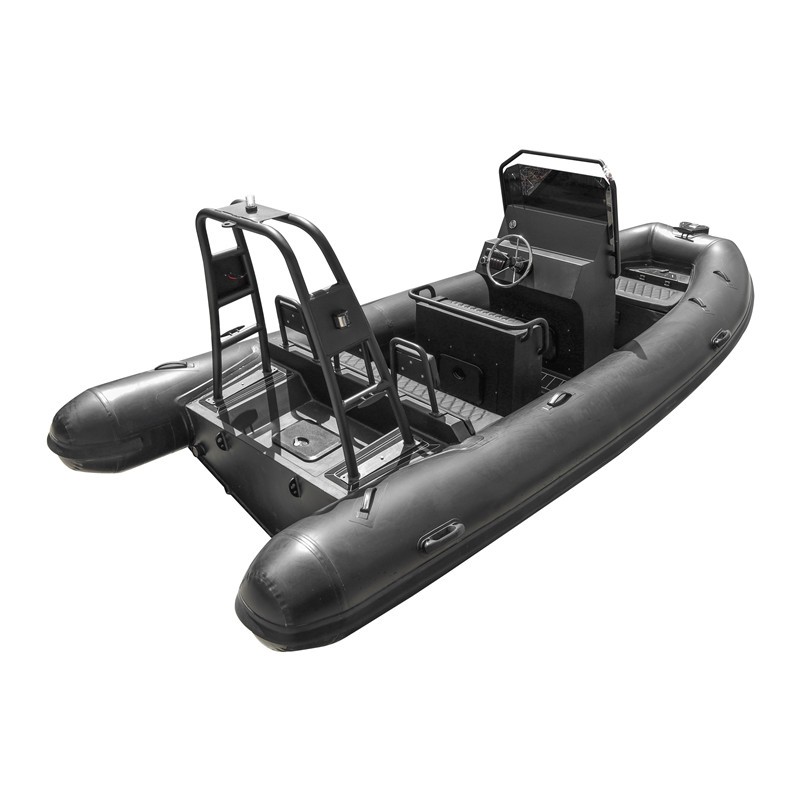The image features an inflatable, military-style speedboat against a plain white background. The boat, primarily in shades of black with a shiny silver steering wheel, suggests a compact but robust design suitable for tactical operations, similar to those used by Navy SEALs. It seats about four people and has a rugged inflatable raft-like exterior encompassing the vessel, equipped with handles along the sides and top for stability and easy access from the water. The boat includes a steering console with a protective darkened glass and a roll cage bar at the back which might support additional equipment such as a light. Additionally, there are seating areas with bars providing structural support and headrests, and a small storage compartment with a lid. The boat's design and build emphasize functionality and resilience, suitable for high-speed maneuvers and potentially rough conditions.